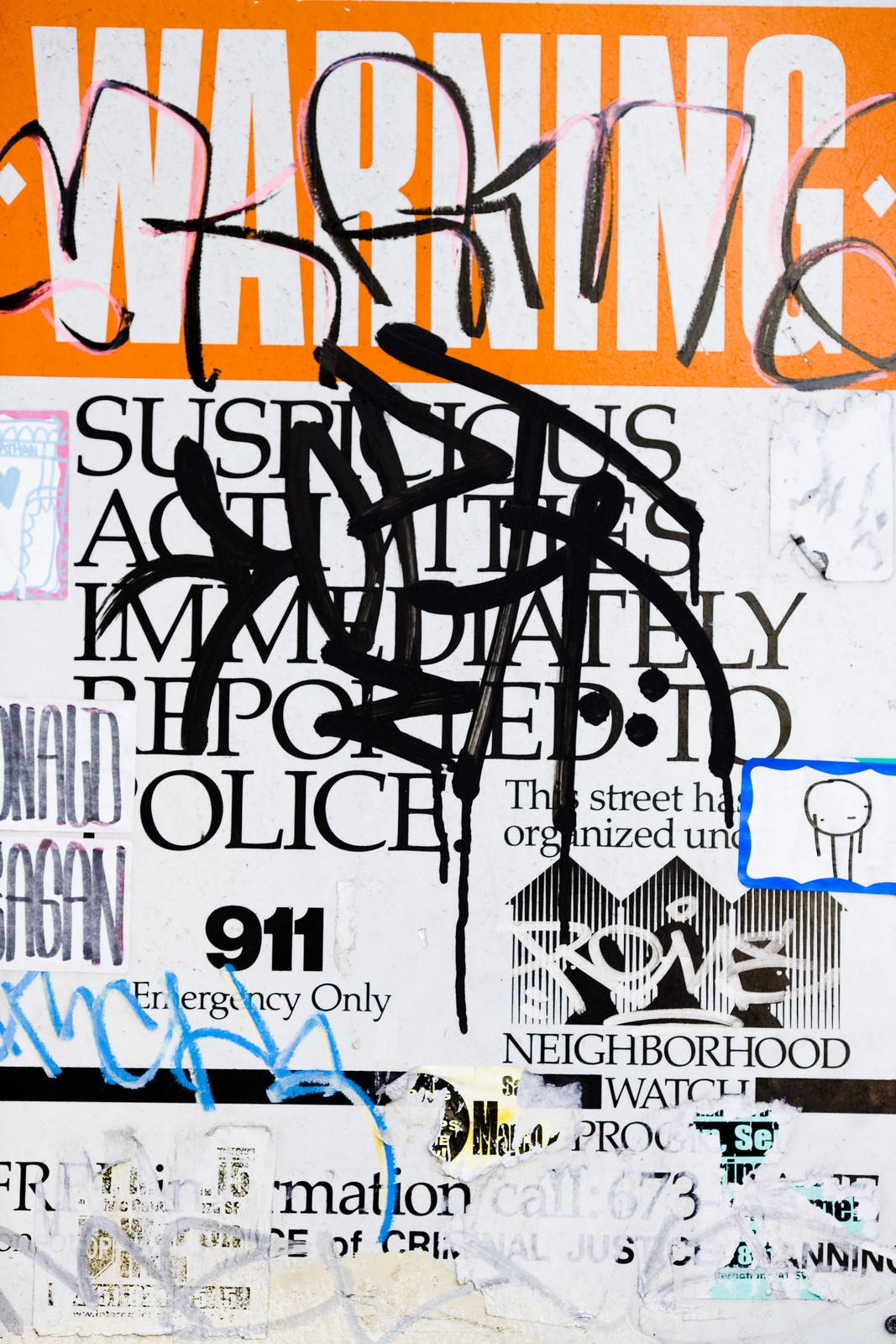The image depicts a heavily vandalized sign originally intended for a neighborhood watch program. The sign, featuring large white letters on an orange background, reads "Warning" at the top. Below that, in white text, it states "Suspicious activities immediately reported to police," and towards the bottom, it indicates "911 Emergency Only." The message also mentions that the street is organized under a neighborhood watch program. 

However, the sign has been defaced extensively. The word "Warning" at the top is almost obscured by thick marker scribbles. The central message about reporting suspicious activities is heavily crossed out with black marker, making it difficult to read. Additionally, on the left side and lower parts of the sign, there are various other markings and graffiti in black, baby blue, and light gray. Some of this graffiti includes illegible symbols and letters that might resemble an arrow, a P, and a T. The sign itself is torn at the bottom, adding to its rough and chaotic appearance, and there are attempts to clean some of the graffiti that were unsuccessful, leaving the lower parts especially difficult to decipher.